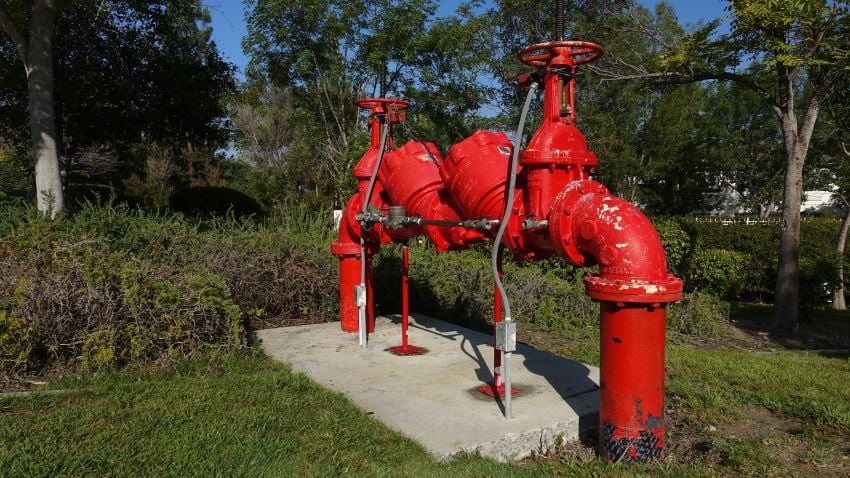The photograph is an outdoor daytime scene featuring a vivid grassy hillside under a deep blue sky with no clouds. Centered prominently are large, bright red pipes emerging from a stone block placed at a slant, with the closest corner in the lower left and the farthest in the upper right of the image. These pipes form a half-U shape and are adorned with valve controls resembling steering wheels positioned at the top. Two smaller pipes connect to the larger main pipe, all framed by additional gray electrical cords that feed into a power box at the base. The scene is surrounded by vibrant green grass, trees, and bushes, suggesting an environment akin to an orchard, with even a hint of a garden to the left. In the background, there are glimpses of white buildings, possibly houses, partially obscured by the lush foliage. This arrangement suggests an irrigation system, complex and substantial in size, set against the serene natural backdrop.